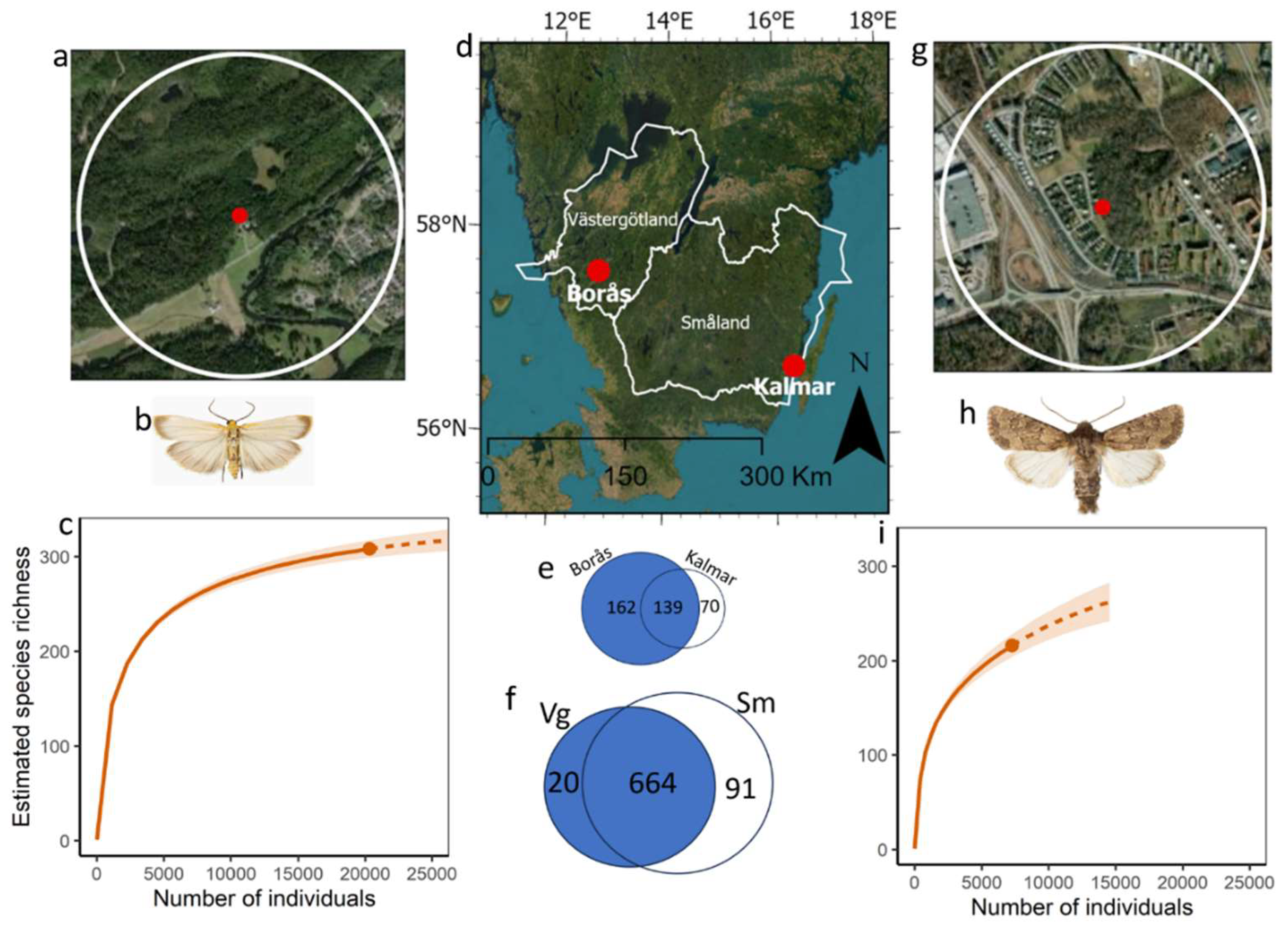This illustration comprises six distinct panels, each identified by a specific letter from A to H, presenting a comprehensive visual survey of moth species populations and their distribution across various regions.

- **Panel A** (top left corner) features a satellite view of a geographic region, marked by a red circle centered within a larger white outlined circle.
- **Panel B** (below A) shows an image of a moth with white and tan coloring.
- **Panel C** (to the right of B) is a chart that plots "Estimated Species Richness" against "Number of Individuals" with a prominent red line.
- **Panel D** (top middle) illustrates another map, likely of Sweden, showing cities such as Västra Gotland, Borås, and Smaland, and is marked by degrees along the sides and top.
- **Panel E** (top right) displays a blue circle with a partially white circle labeled "boros" and "calamar".
- **Panel F** (also larger and dark blue, next to E) features another partially white circle marked "VG" and "SM".
- **Panel G** (top right corner) provides an additional map view with a white circle and a red dot.
- **Panel H** (below G) depicts another moth, with a white and brown coloration.
- **Panel I** (below H) is a second chart indicating the "Number of Individuals" with an increasing red line.

Letters B and H both show images of different moth species, whereas letters C and I represent charts detailed with population data. The central images (D, E, F) focus on the geographical distribution overlapping with the regions where the moth populations have been studied. This illustration offers a detailed and systematic depiction of the species richness and distribution of multiple moth populations across these mapped areas.